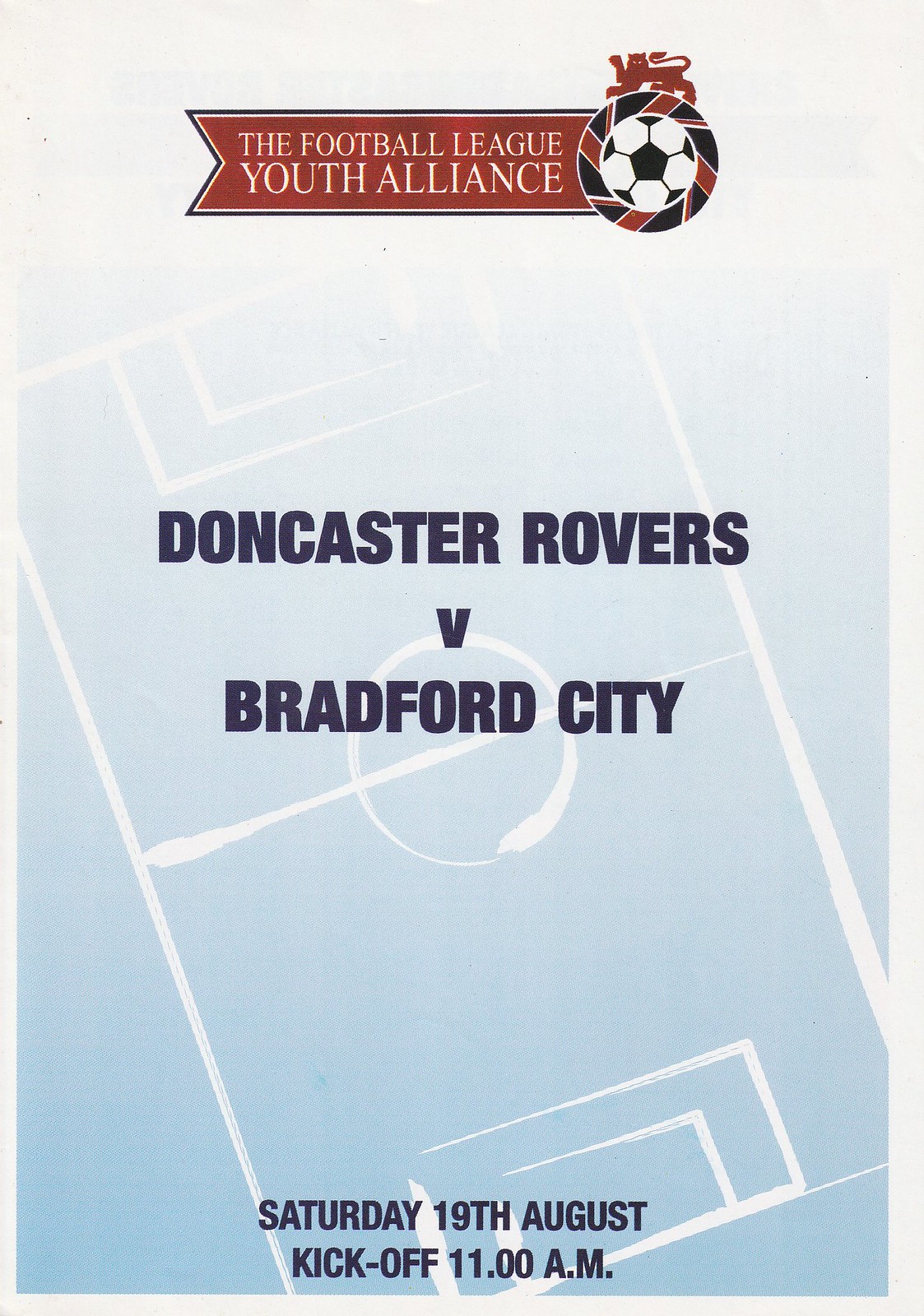This image, resembling the front cover of an old magazine or newspaper edition, is rectangular and taller than it is wide, set against a blue background with a light-colored border. At the top, a soccer ball is depicted with a white background, encircled by alternating black and red stripes. Overlaying this is an image of a red lion. Extending left from the soccer ball is a red banner with a black outline, containing white text that reads "The Football League Youth Alliance."

Beneath this, a simple illustration of a white soccer field is drawn against the blue background. Centered over this, in dark navy blue or black text, are the words "Doncaster Rovers versus Bradford City." At the bottom center, the caption reads, "Saturday 19th August, kickoff 11 o'clock a.m."